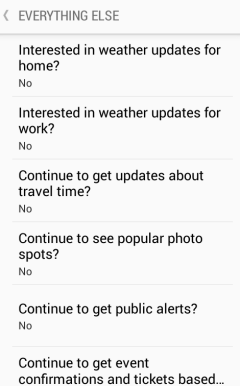Here is a cleaned-up and detailed caption for the image described:

"A screenshot of a website settings menu, possibly part of a Q&A system, displaying various notification preferences. The interface features a clean design with black text on a white background and gray lettering at the top alongside a back arrow. The options listed allow the user to control different types of notifications they receive, including updates about weather from home and work, travel time notifications, popular photo spots, public alerts, and event confirmations. All options have been set to 'no,' indicating that the user does not wish to receive these notifications. The text and options appear in the order mentioned."